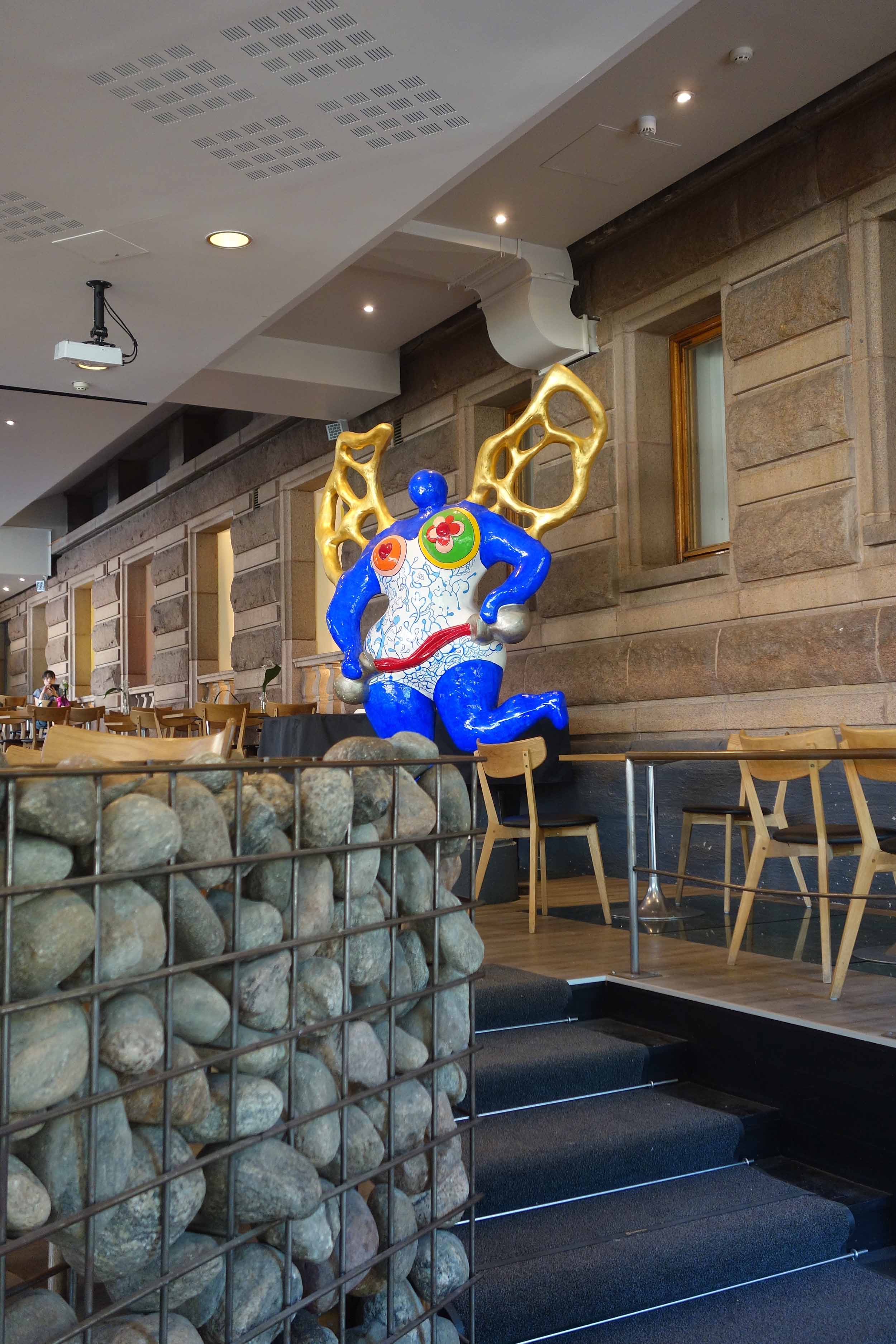This image captures the interior of a uniquely designed restaurant. Central to the scene is a visually striking statue perched atop a container filled with rocks held in place by a metal grid, giving the impression of a rock wall. The statue depicts a faceless blue figure, adorned in an electric blue bodysuit with an unmistakably feminine chest. She is equipped with golden abstract wings and holds a bent barbell in her hands. Detailed elements of her attire include hints of orange armor on one side and potential green or blue on the other. Surrounding her, the dining area is set on a higher level accessible by a short flight of carpeted stairs. The restaurant features a mix of tables and chairs with light wood and dark seats. The walls have a rustic, lumber-like appearance, contributing to the cozy ambiance with their brown and tan stones. A projector is noticeable on the white ceiling, and a distant figure can be seen seated among the diners, completing this snapshot of a captivating, art-infused dining environment.